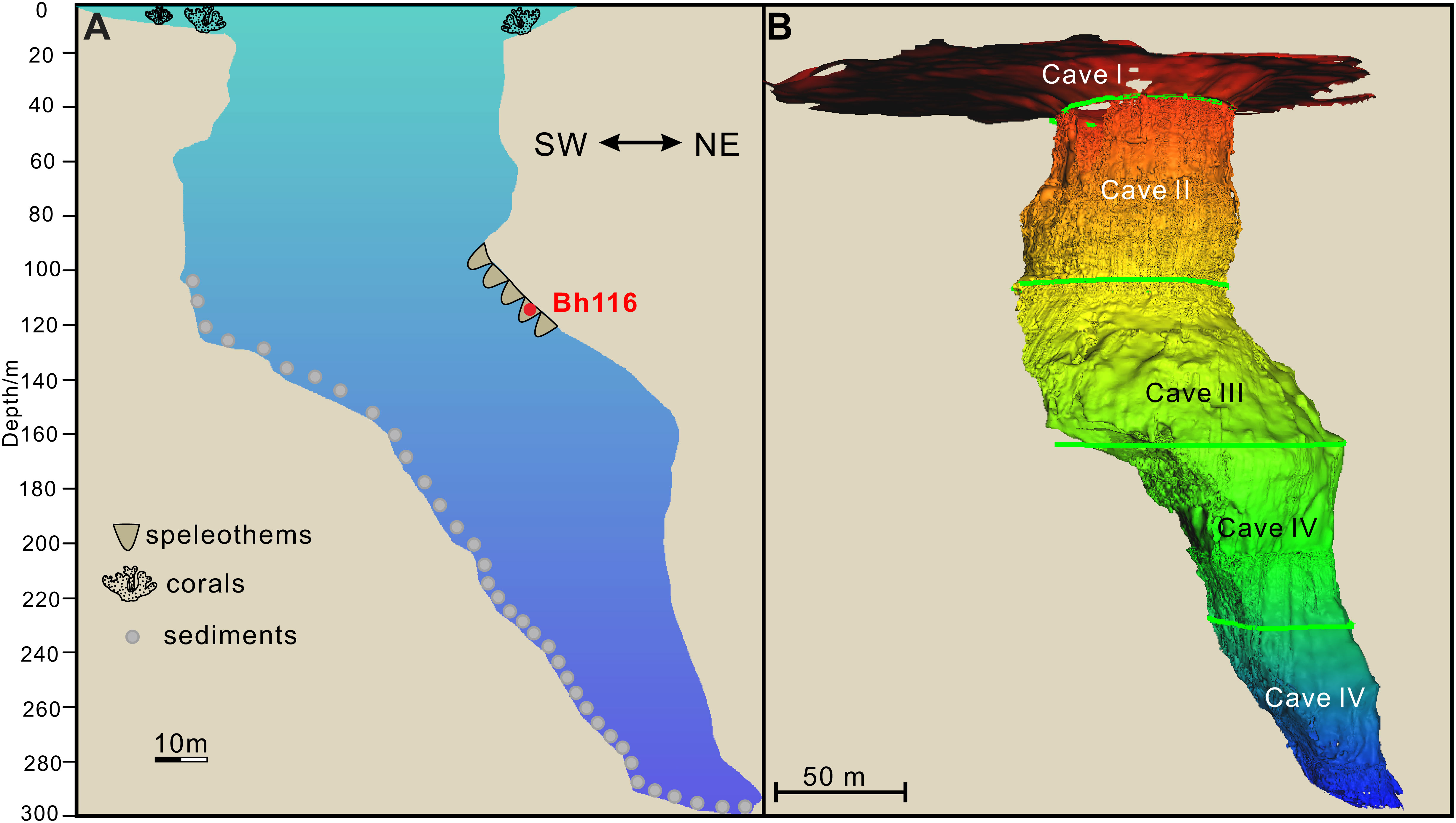The image consists of two side-by-side sonar readings of a cave, labeled A and B. On the left, in section A, the cave is depicted with gradations of blue, ranging from light turquoise at the top to deep blue and purple at the bottom. The cave's shape resembles the state of California and features depth markers on the left side, extending from 0 to 300 meters. Arrows indicating SW (southwest) and NE (northeast) direct across the middle of this section, along with a red marker labeled BH116.

Section B, on the right, presents a more detailed and colorized version of the same cave. This image is segmented into distinct layers: CAVE1 in red at the top, followed by CAVE2 in orange, CAVE3 in yellow transitioning to lime green, CAVE4 in dark green, and CAVE5 in blue and purple at the bottom. Each cave section is labeled with Roman numerals. A legend at the corner of section B categorizes different features, such as speleothems, corals, and sediments. The cave's depths and structure are conveyed with texture, providing a vivid and detailed representation of the cave's stratified composition. Both sections are labeled accurately to enhance the understanding of the cave's anatomy.